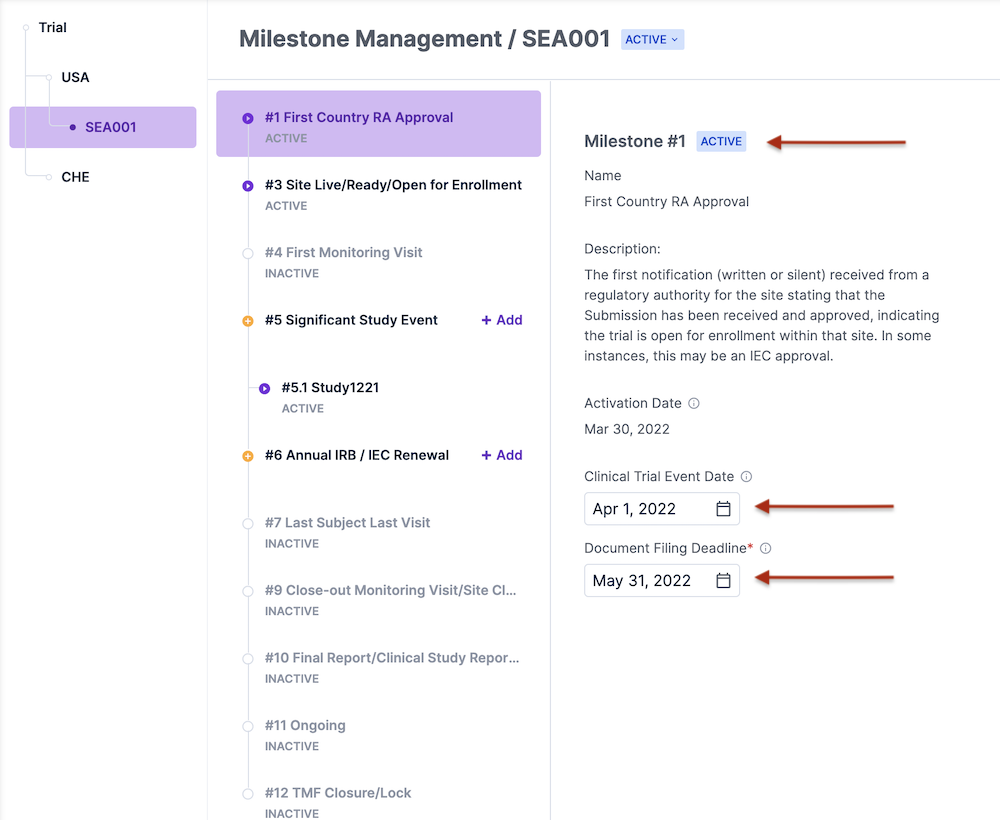The web page features an abundance of information related to Milestone Management, labeled with the identifier CEA001. At the very top, there is a text header in black that reads "Milestone Management / CEA001." Beside this header, there is an interactive element: a button styled with blue text on a light blue background, featuring a small down arrow, indicating that it is clickable.

To the left of the central content, it lists "Trial" with "USA" directly below, followed by the label "CEA001" and underneath that "CHE." 

The main body of the page is densely packed with listed information. At the top of the main content section, it refers to "Number one, first country, RA approval." This is followed by details presented in a sequential list: 
1. First Country, RA Approval 
2. Site, Live, Ready, Open for Enrollment (labeled as number three)
3. First Monitoring Visit (labeled as number four)
4. Significant Study Event, with an option to add details.

Continuing downward, some of the text appears grayed out, suggesting less importance or a disabled state. On the right side, bold black font indicates "Milestone number one, active," accompanied by a red arrow pointing left towards the active button mentioned earlier. Below this, there is a field labeled "Name, first country, RA approval," followed by a small description, an activation date, and a series of dates ranging from April to May.

This comprehensive layout and detailed labeling provide a clear overview of the milestones and study-related events, designed to facilitate the management of clinical trials.